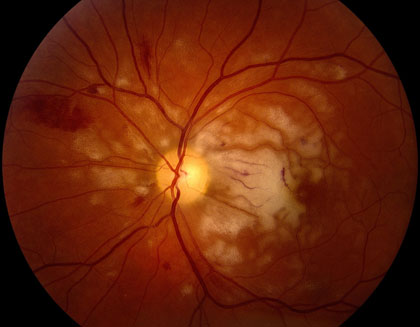The image showcases a zoomed-in view of what appears to be living tissue, set against a black background creating a stark contrast. The central focus is a pale yellow, almost orange, spherical shape, surrounded by a larger pale red sphere. This larger sphere is detailed with dark red veins and smudge-like marks, giving it a textured appearance with occasional bumps. The intricate network of dark red lines crisscrossing over the surface suggests the likeness of veins or nerves, adding a scientific and organic feel to the composition. The vivid yellow center, standing out brightly, adds another layer of complexity and visual interest to the image.